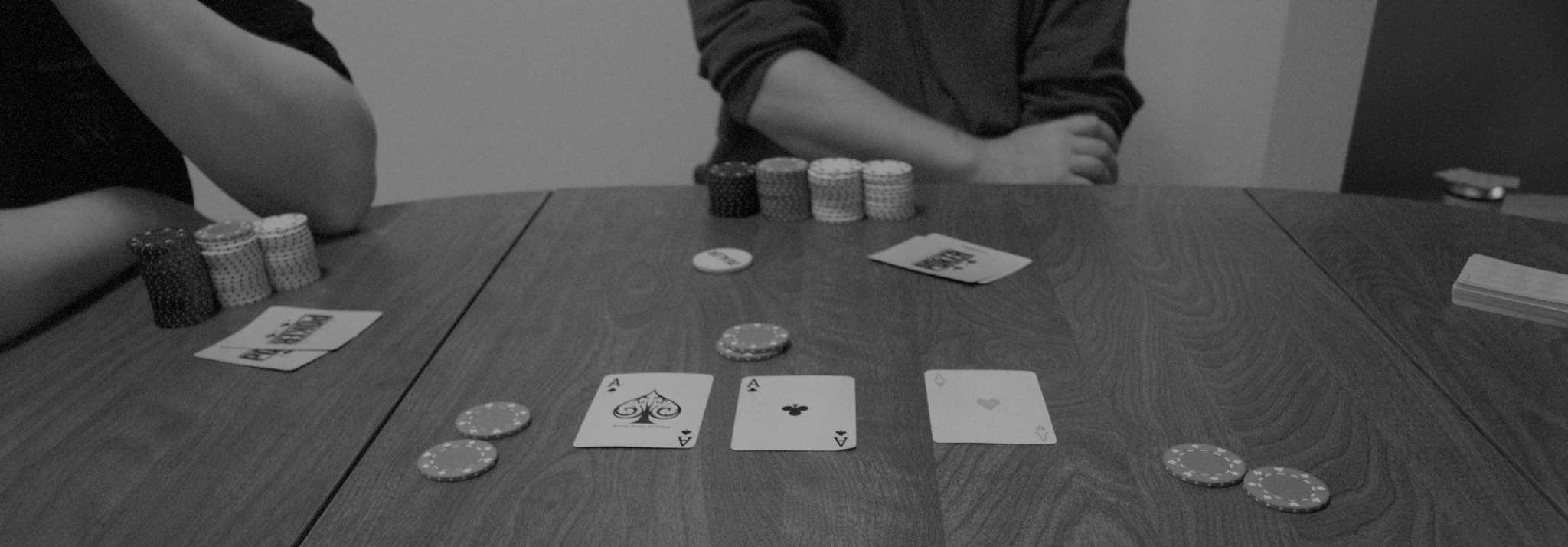This black-and-white photograph captures an intimate indoor setting of a card game in progress. At the center of the scene, a wooden table, discernible by its grain and texture despite the monochrome palette, hosts the game. Three individuals are seated around the table, engaged in a round of blackjack. 

The center player appears to be dominating the game, with a considerable stack of poker chips in front of them, suggesting their winning streak. This individual is identifiable by their elbows resting confidently on the table. To their left, another player, dressed in a dark-colored shirt, sits with their arms folded, perhaps contemplating their next move or reconsidering their strategy. The third participant, positioned to the right, remains less distinguishable but is equally engrossed in the game.

Scattered on the table, a variety of poker chips, distinguishable by the different shades of gray, indicate the competitive nature of the game. The dealer's hand is visible, showing the two of spades and the six of diamonds, alongside an additional card that remains partially obscured. The players' cards, however, stay hidden from view, adding an element of suspense to the scene.

Despite the limitations of the photograph's size and color, the composition vividly conveys the tension and camaraderie of the moment, each player's stance and chip count hinting at their respective fortunes in this round of blackjack.